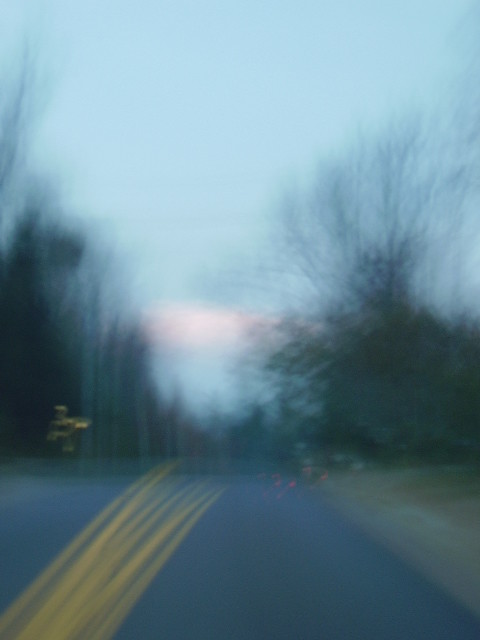A blurry photograph captures a street scene during the ethereal transition of dusk. The image, though lackluster in sharpness, reveals a road characterized by two solid yellow lines demarcating the lanes, creating an illusion of multiple lines crisscrossing due to the blur. Patches of grass flank the sides of the street, adding a touch of nature to the urban setting. In the distance, the faint, red glow of brake lights hints at a car slowing down or pausing. The roadside is home to large, skeletal trees, barren of leaves, which stand tall against the evening sky, now tinged with a delicate pink hue from the setting sun. On the left-hand side of the road, a yellow traffic sign, though indistinct, adds to the scene's authenticity with its familiar presence.